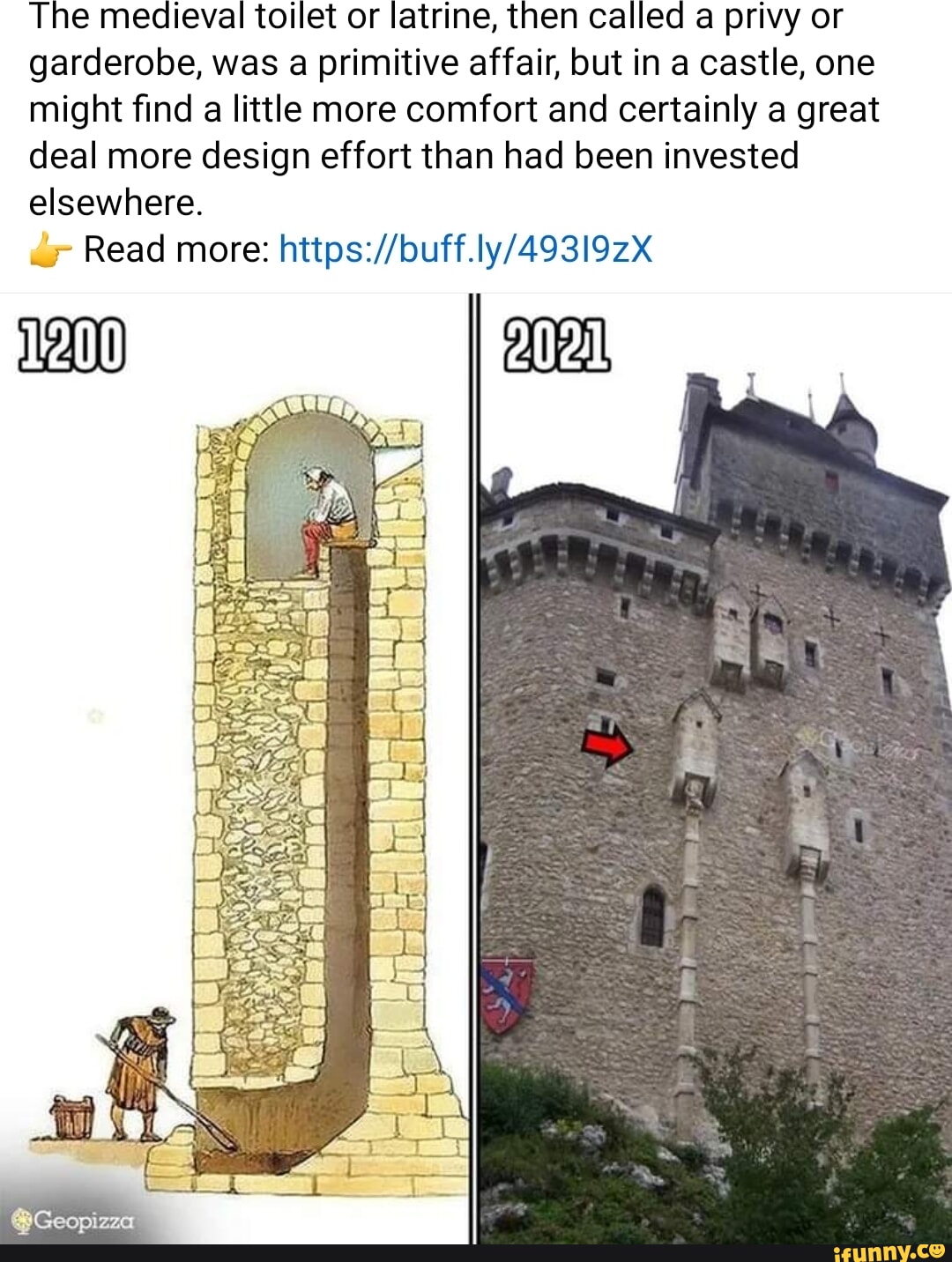This image is a side-by-side comparison featuring medieval and modern depictions of castle toilets. On the left side, an animated cross-section diagram labeled "1200" illustrates a medieval toilet or latrine, also called a privy or garderobe. In the diagram, a person is shown using the toilet at the top of a castle turret, where waste is seen falling through a chute downwards to the ground level, where another person is depicted scooping it away with a long-handled tool. The right side of the image shows a photograph labeled "2021," depicting a modern-day castle with structures jutting out, likely the same medieval toilets shown in the diagram. At the top of the image, text reads: "The medieval toilet, or latrine, then called a privy or garderobe, was a primitive affair, but in a castle, one might find a little more comfort and certainly a great deal more design effort than had been invested elsewhere." A finger emoji points to a "Read more" link. The image appears to be a screenshot of a tweet and credits Geopizza and iFunny.co.